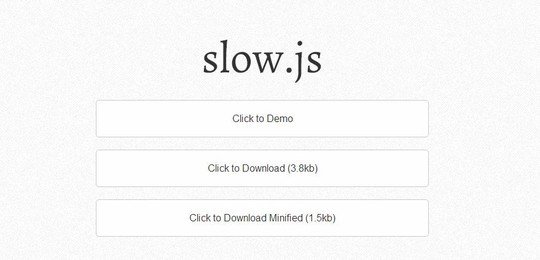This image is a screenshot showing a minimalistic portion of a web page with a predominantly white background and very light gray accents, nearly blending into the white. The text on the page is a dark gray, aiding readability. Centered prominently at the top is the word "slow.js," indicating a reference likely related to JavaScript.

Below the title "slow.js," three outlined rectangles are aligned vertically, each bordered by very thin, light gray lines. These rectangles serve as interactive buttons:

1. The first rectangle contains the text "Click to Demo" in gray font, suggesting a link to a demonstration.
2. The second rectangle reads "Click to Download (3.8 KB)," indicating a small file available for download.
3. The third rectangle says "Click to Download minified (1.5 KB)," denoting a compressed version of the file for download.

Each button is clearly labeled with its function, providing options for users to interact with the web content.